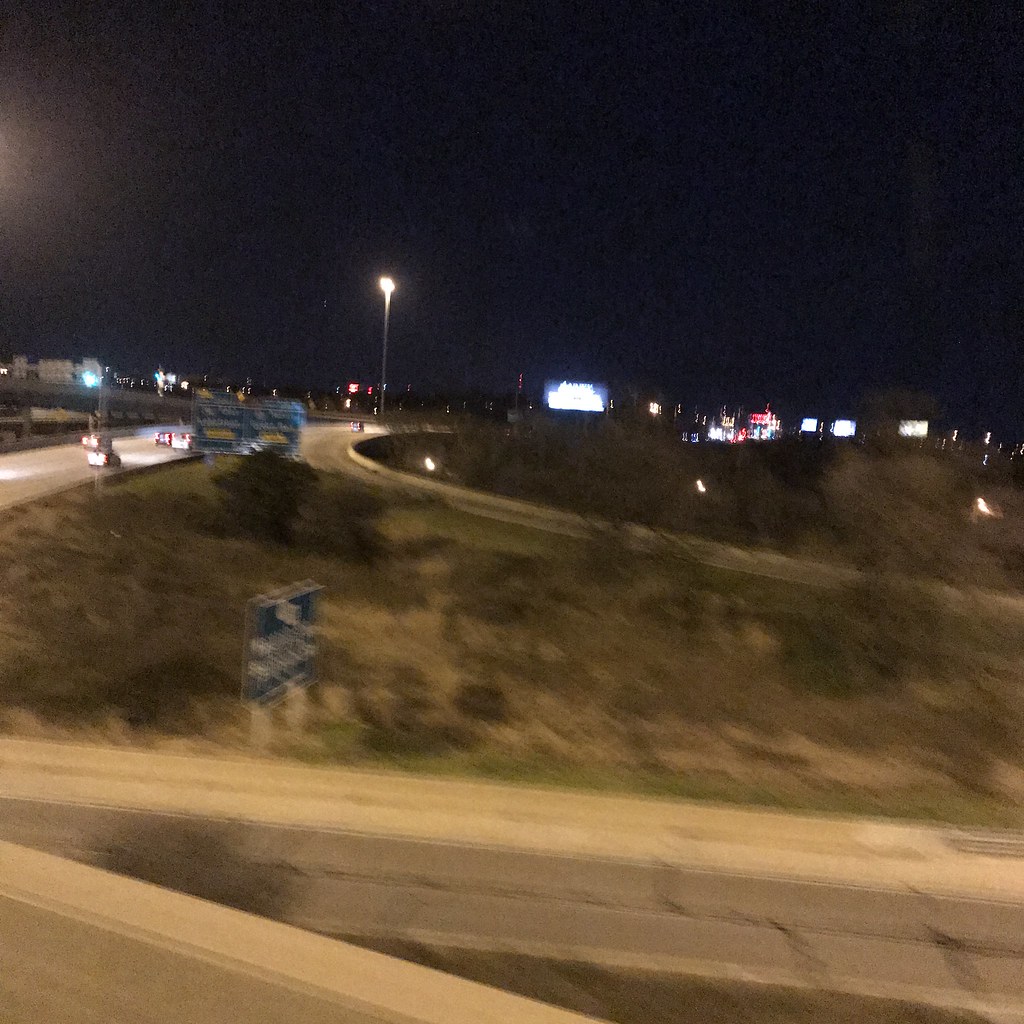A nighttime photograph captures a complex highway interchange. Dominating the foreground is a four-lane highway, though it appears slightly blurry and might actually be two lanes; the roadway is a tannish color. Adjacent to the highway stands a street sign with a blue back, though the text is indistinct due to the image's blur. A grassy median populated with scrub brush and greenery lies next to the road. Beyond this area, an entrance or exit ramp curves into view, originating from the right and sweeping upward towards the middle of the image before blending into the main traffic flow. Several high-mounted blue signs provide guidance to drivers as they navigate this curved ramp. Once on the ramp, a series of illuminated signs with red and white lettering become visible, guiding vehicles onward. The night sky forms a dark, black, and gray backdrop to the scene. A tall pole lamp towers above the entire interchange, casting a bright white light and revealing the intricate details of the freeway below.